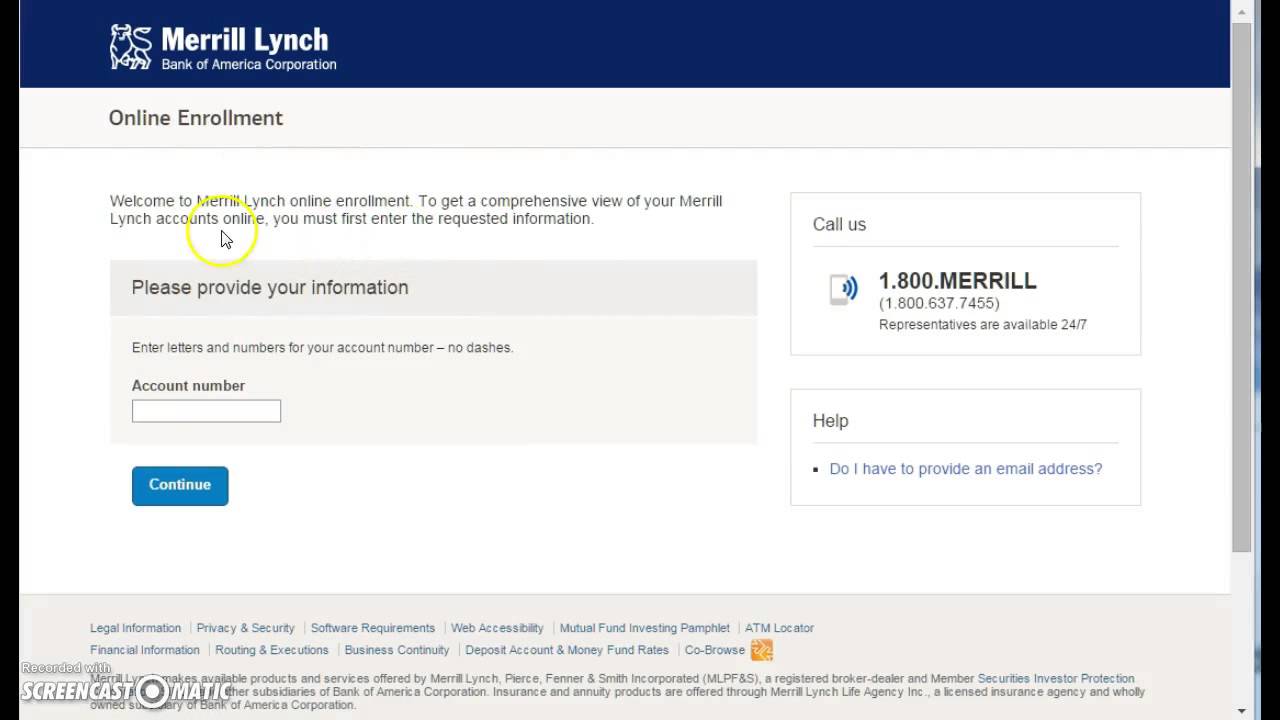This screenshot captures the online enrollment page for Merrill Lynch, a brokerage firm under the Bank of America Corporation. The design features a dark navy blue banner set against a white and gray background. The page welcomes users to Merrill Lynch Online Enrollment, directing them to enter their account information to gain comprehensive online access to their Merrill Lynch accounts. Specific instructions prompt the user to input their account number, explicitly stating to enter letters and numbers without dashes in the provided dialog box. Upon entering this information, the user can select a 'Continue' option to proceed, likely leading to additional steps in the enrollment process.

On the right-hand side of the screen, a taskbar displays Merrill Lynch's customer support contact number, 1-800-MERRILL (1-800-637-7455), with a note that representatives are available 24/7 to assist. Additionally, a help section addresses common questions, including whether an email address is required for the enrollment process. The layout is designed to guide users through enrollment efficiently while providing accessible support options.